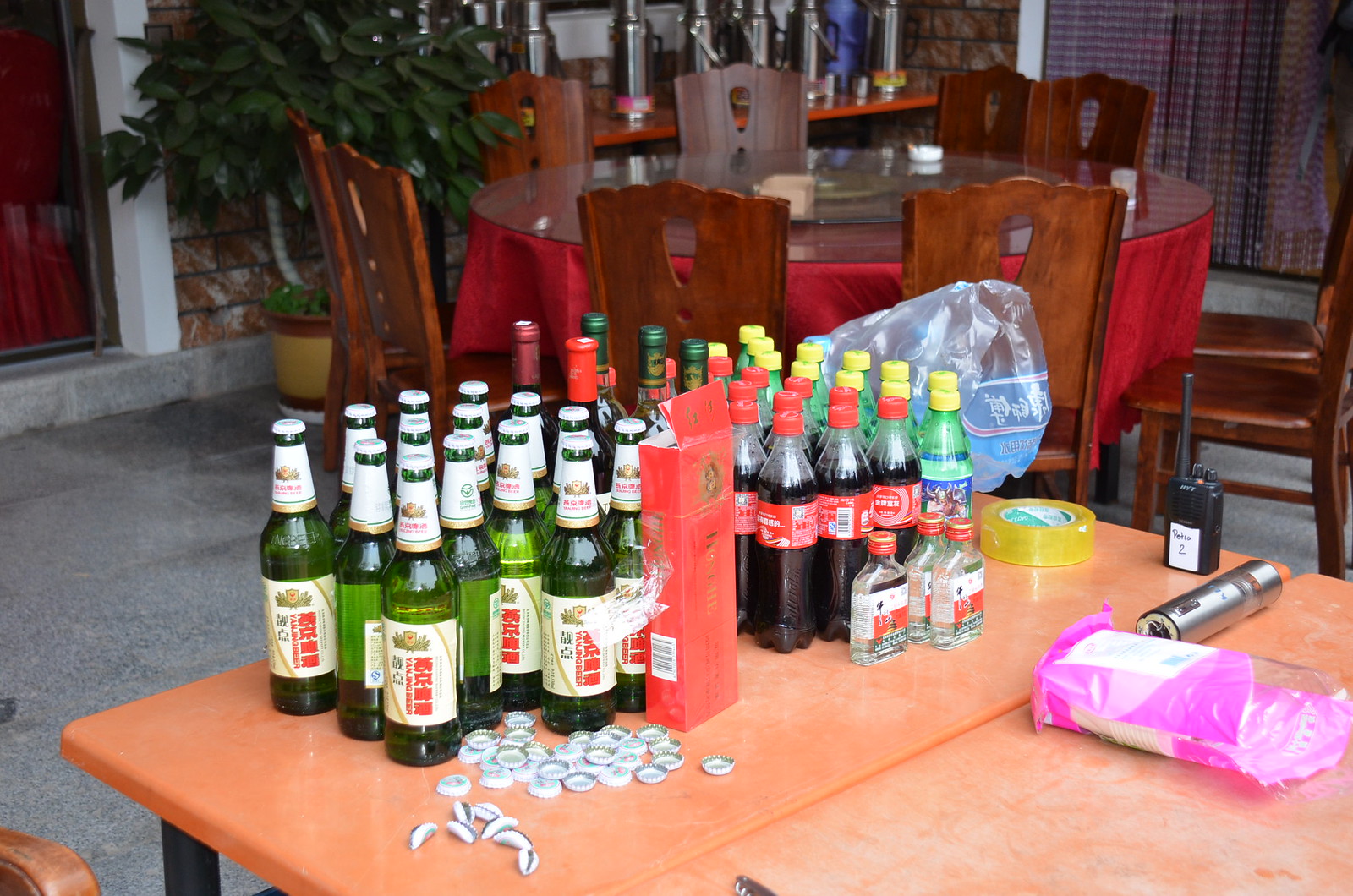In the outdoor photograph, the main focus is an orange plastic folding table laden with an assortment of bottles and other objects. To the left side of the table are neatly arranged rows of 13-14 green glass beer bottles, identifiable as Yanjing beer, with a cluster of white bottle caps, some of which are crushed or folded in half, in front of them. To the right of these beer bottles are various soda bottles, including clear plastic bottles with red labels and caps, reminiscent of Coca-Cola but without the brand name, and clear green plastic bottles with yellow caps resembling Sprite. Adjacent to these soda bottles is a roll of yellow tape and a walkie-talkie, which is flanked by a gray cylindrical object and a pink and white plastic bag positioned slightly to the left.

In the background, there is a round dining table with a glass top and a red tablecloth beneath it, surrounded by ten dark wooden dining chairs arranged in a circle. Further back, another table holds carafes of coffee. The setting appears to be an outdoor patio with concrete flooring, and the bottles, featuring Asian — likely Chinese — lettering, hint at a cultural context.